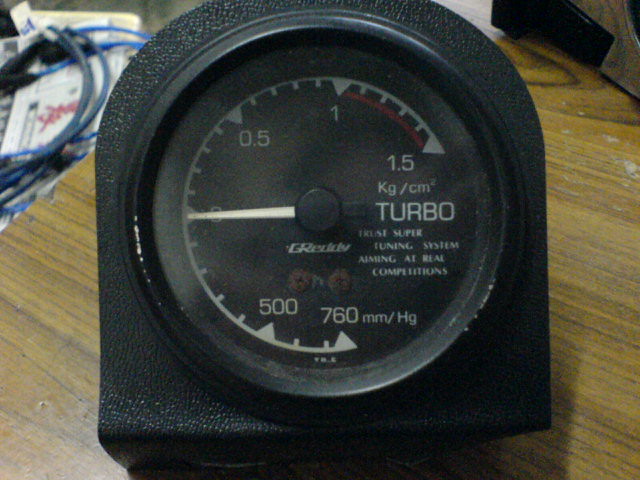This image features a pressure gauge encased in a black, round housing resembling a clock face. The face of the gauge is entirely black, including the rim, enhancing its sleek appearance. This dial prominently displays numbers and text; at the bottom, the numeral "760" is marked, while at the 2 o'clock position, the value "1.5" is visible. Beneath this, the unit of measurement is specified as "kg/cm²," followed by the word "Turbo" in bold text. The gauge has a single hand, which currently points to the 9 o'clock position. Additionally, more precise markings are noted, such as "760" at approximately the 5.25 o'clock mark, "500" at 5.35, "0.5" at 11.50, and "1" at 12.05. The pressure gauge is set on a wooden table, with an assortment of wires situated behind it, suggesting a connection to a broader mechanical or electrical system.